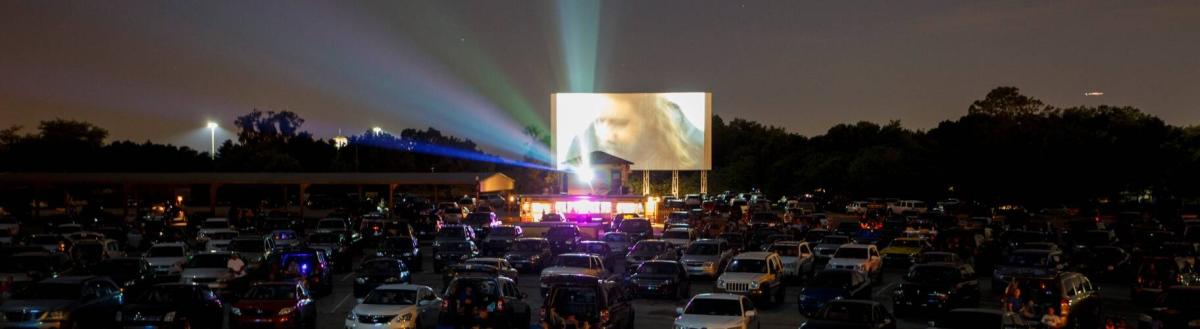This panoramic, rectangular color photograph captures the nighttime scene of a drive-in movie theater. The slightly elevated image presents a wide, narrow view that showcases a large, glowing screen positioned prominently in the middle ground. A blurry image of a person's face is projected onto this screen, adding to the cinematic atmosphere. Below the screen, a brightly lit concession stand draws attention with its illumination. In front of the screen, numerous cars are parked in neat rows, filling the lower half of the photograph. To the left side, there is a covered area adjacent to the projector booth, which is shining a powerful beam of light towards the screen, creating an iconic drive-in movie theater feel. The background features a silhouette of trees and faint street lamps lining the horizon, while the night sky, predominantly dark with perhaps one visible star, encapsulates the serene ambiance of an outdoor movie night.